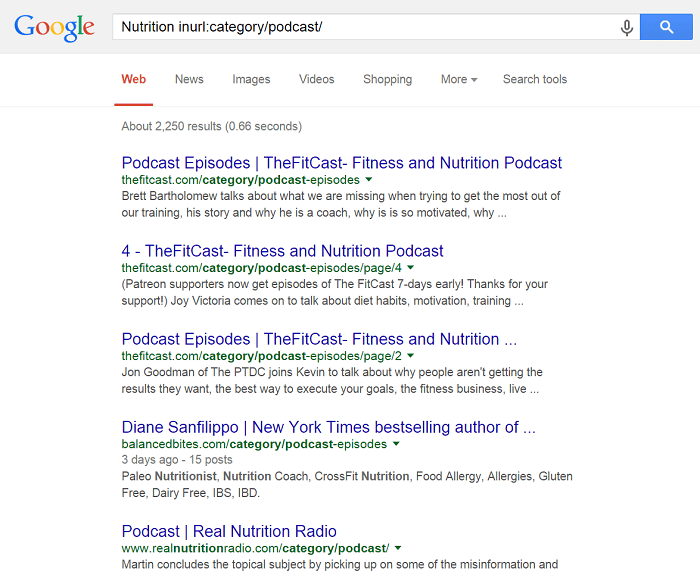This is an image showing a screenshot from the Google website. In the top left corner, the iconic multicolored "Google" logo is prominently displayed with hues of blue, red, yellow, and green. Adjacent to the logo is a search bar featuring a white background. Within this search bar, in black text, reads “nutrition INURL:category/podcast/”. To the right of the search bar, there's a small microphone icon and a blue rectangle containing a white magnifying glass symbol, indicating the search button.

Below the search bar are various categories for filtering search results, listed as "Web," "News," "Images," "Videos," "Shopping," "More," and "Search tools." Among these options, "Web" is selected, highlighted in red with an underline, while the others remain gray.

The search results section displays five different entries, and above them, it is noted that there are "about 2,250 results" in gray text. The top result is titled "Podcast Episodes: The Fitcast: Fitness and Nutrition Podcast," written in blue text. Below this title, there is some additional information in gray text.

Following that, the second listing repeats a similar title: “The Fitcast: Fitness and Nutrition Podcast,” again accompanied by pertinent information beneath in gray. 

The third result features "Diane Sanfilippo, New York Times Bestselling Author" with further details following it.

Finally, the fifth result is titled "Podcast: Real Nutrition Radio" and, as with the previous entries, includes supplementary information below it in gray text.